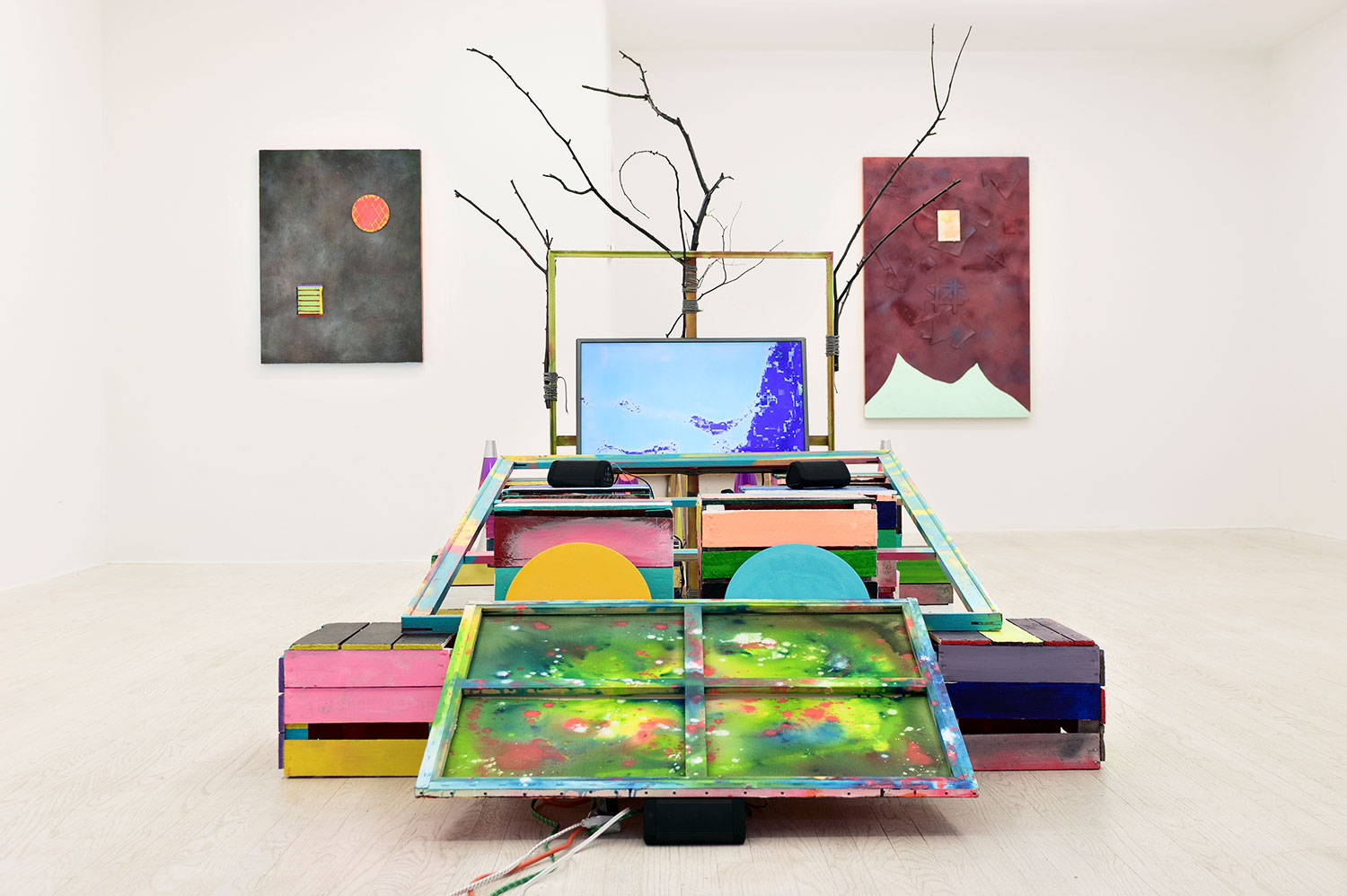The image depicts a vibrant and intricate art installation set in a gallery with white walls and a pale wooden floor. On the left wall, there is a rectangular canvas painted with a black smoky gray hue, featuring a red circle and a green square. Adjacent to it, on the right wall, is a terracotta brown canvas accented with a yellow square in the center and white paint splatters. Below this brown canvas, there appears to be a landscape silhouette in a pale green color. The centerpiece of the gallery is an abstract structure resembling a makeshift car, composed of stacked wooden pallets, spray-painted and splattered with multiple colors—green, yellow, white, and red. This structure includes window frames or the back of canvases splattered with paint, placed atop the wooden steps painted in shades of pink, purple, yellow, and teal. In the middle of this installation, larger frames and canvases with blue and green backgrounds showcase abstract designs. The floor also features semi-circular shapes, mimicking the appearance of half-plates, one yellow and one blue. Completing the scene, a bare tree branch is visible through an empty frame connected to the installation, adding an organic touch to the eclectic array of colors and forms.